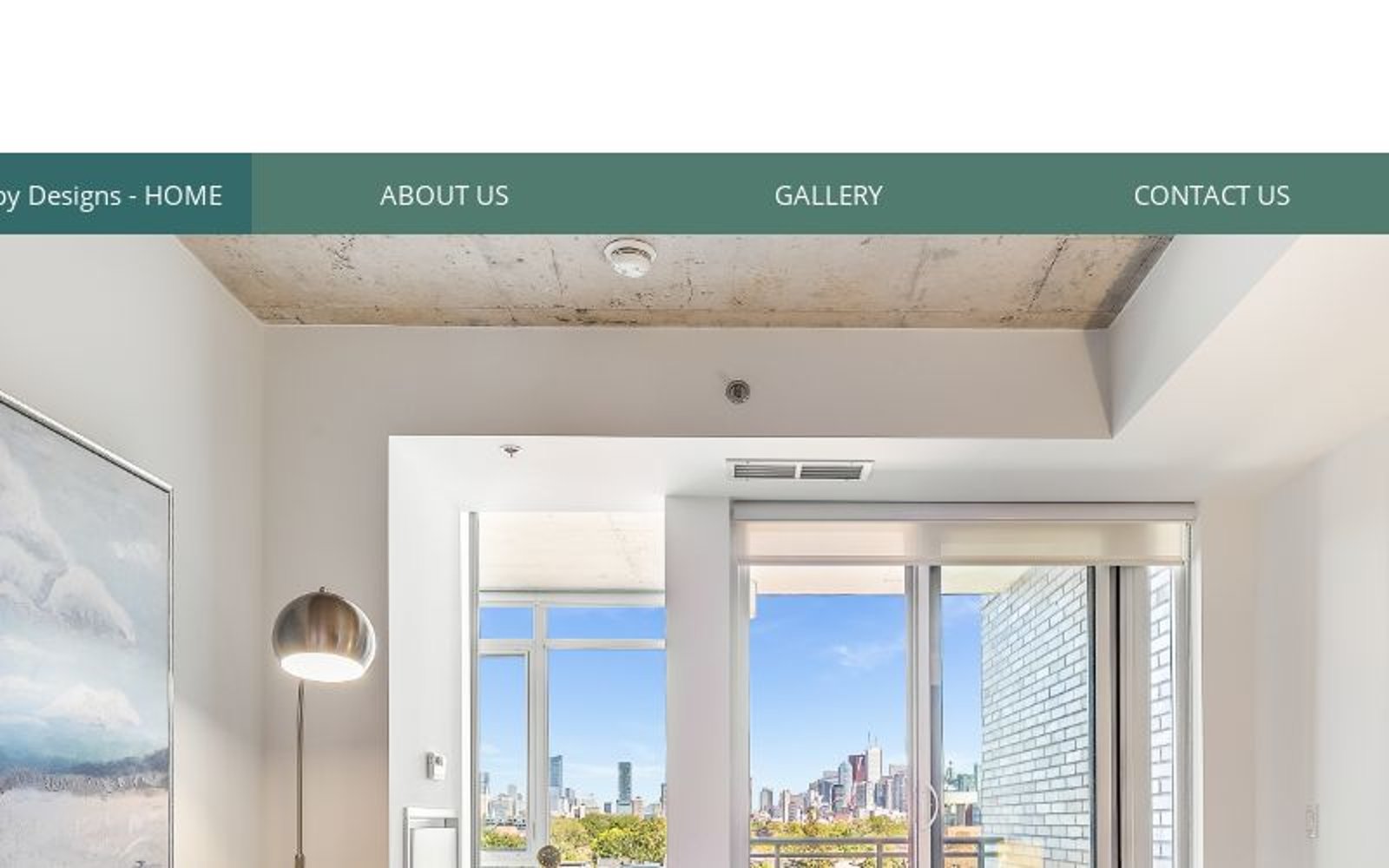A screenshot from a home design website showcases an unfinished yet promising room. The top navigation bar, a blend of darkish lima bean green with a darker shade highlighting the selected menu, displays options such as Home, About Us, Gallery, and Contact Us. The central image captures a room with a rugged ceiling, indicative of ongoing renovations. Despite this, the room boasts refined elements like sliding doors and an unconventional heating system positioned above one of the doors. The right wall, made of white brick, features a scenic city skyline in the distance under a clear blue sky, with lush hedges accentuating the view. The left wall is adorned with a beach photograph, adding a touch of tranquility. A dome light hangs from the ceiling towards the room's left-middle section, and a temperature gauge appears positioned peculiarly outside the main structure. The overall room design seems to bear the hallmarks of AI design, with some structural choices appearing unconventional.